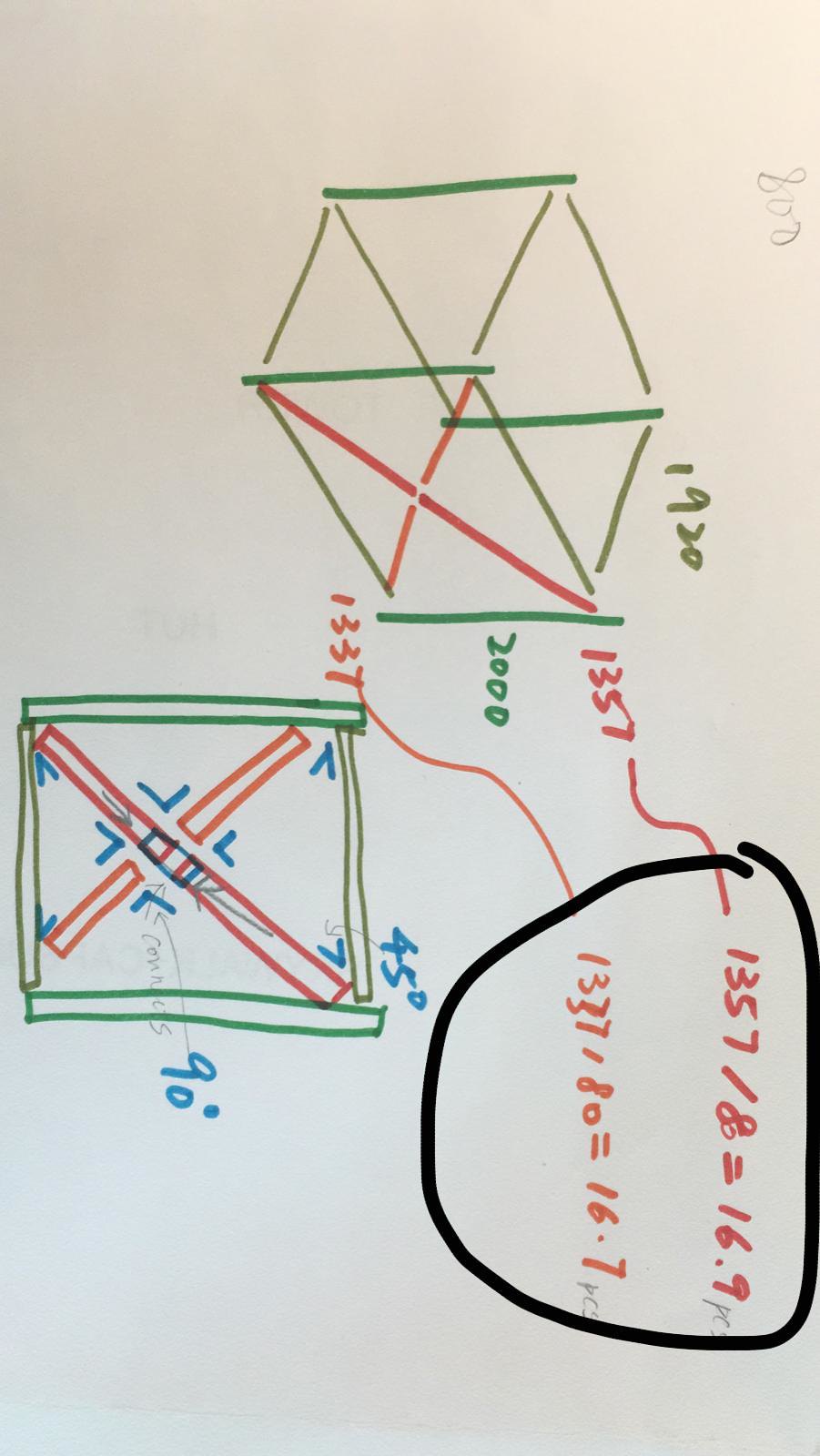The image features a piece of drawing or construction paper, oriented in landscape. Dominated by marker illustrations, it is vividly colorful and complex. In the upper left, a cursive "800" is drawn prominently. Rotating the image reveals a three-dimensional box filled with green, dark green, hints of yellow, orange, and red. The number "1920" is inscribed near the box.

In the upper right portion, there is a black marker notation "1357 / 80 = 16.9" alongside a penciled entry potentially denoting "PCS" or "pieces". Directly below, another calculation "1337 / 80 = 16.7" appears with similar penciled annotation.

Near the middle-bottom of the image, a face-like structure is discernible, featuring an X intersecting with a cube, all framed within rectangles. If viewed in landscape, the main rectangle is likened to a forward slash, with broken segments top and bottom, shaded orange. Another prominent rectangle, this time in red, aligns with the forward slash, while the internal sections blend with blue marker. The outer vertical sides are outlined in green, and the top and bottom rectangles exhibit a yellow-green dark tone.

Notably, in the upper right corner is a notation "45°", and on the right-hand side, another marking reads "90°". A penciled arrow points towards the central angle, indicating a focal measurement or indicating direction related to where the 45° notation resides in the upper right corner.